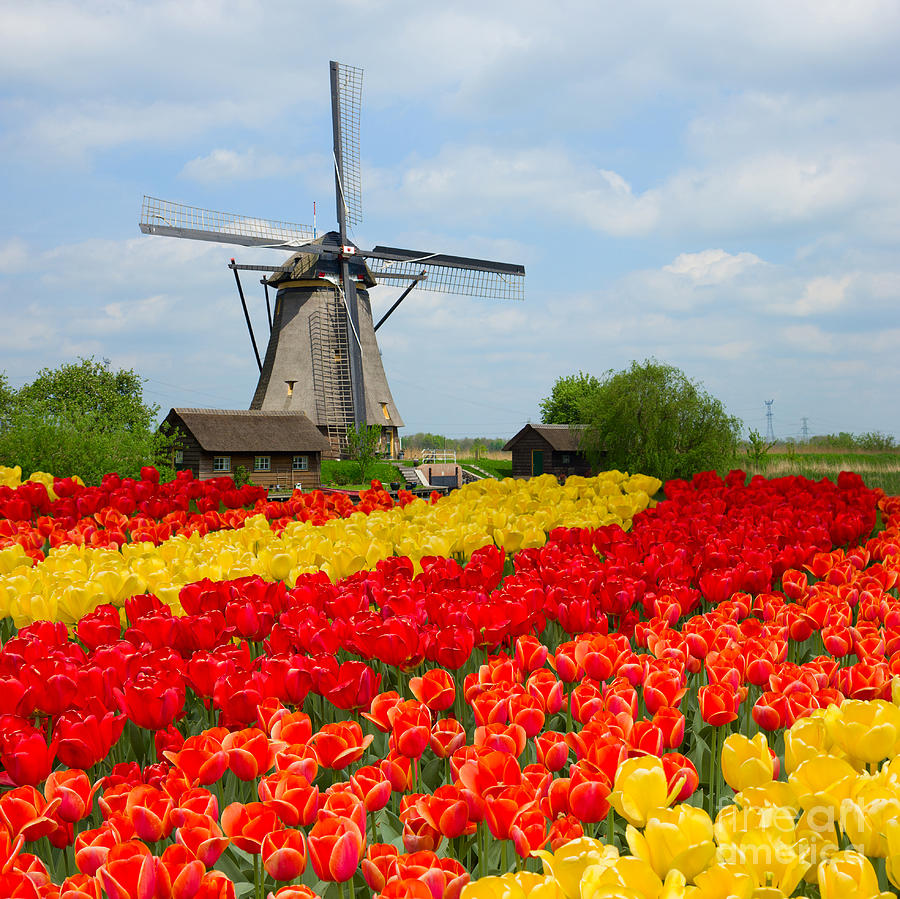The image is a detailed, square-shaped outdoor photograph depicting a vibrant and colorful field of flowers. Rows and rows of bright red, orange, and yellow tulips dominate the lower portion of the image, with green grass interspersed among the blooms. The clarity of the image is striking, capturing the rich hues vividly. In the background, tall green trees are visible, adding depth to the scenery. 

A prominent feature is an old-fashioned, gray windmill near the center of the photograph, characterized by its four mesh-like wings. Flanking the windmill are two quaint, brown log cabins with angled, sloped roofs; the cabin to the left features three small windows. There are additional trees visible near these structures. 

The sky above is a brilliant blue, dotted with a few white clouds, indicating a clear and sunny day. Despite being taken during the daytime, a watermark text is noticed at the bottom right, and the entire setting exudes a serene, picturesque ambiance, perfect for a tranquil country scene.